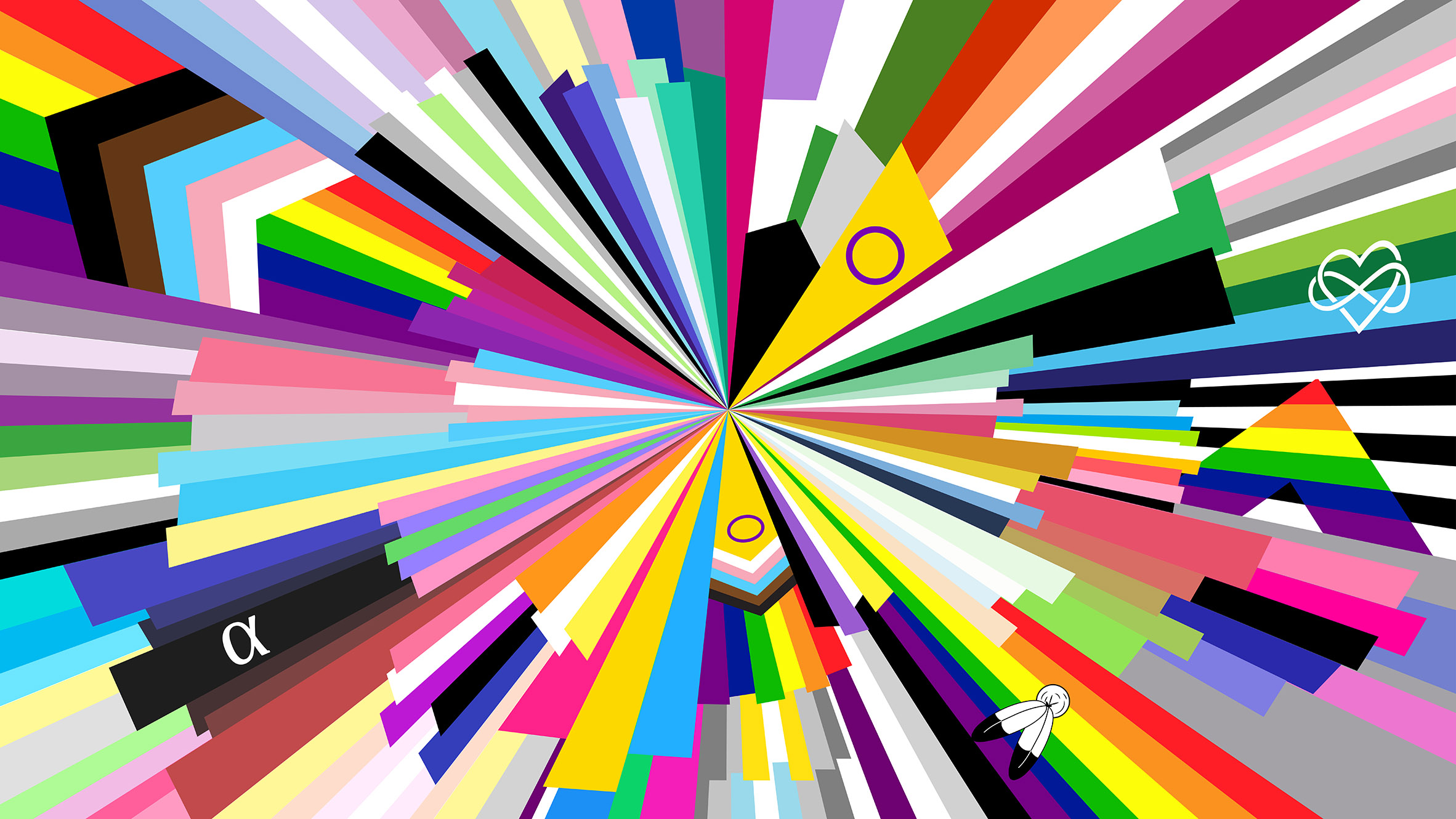This abstract painting showcases an explosion of vibrant colors, resembling a dynamic kaleidoscope. It features a central point from which rays of multiple hues—blacks, whites, various shades of greens, reds, yellows, blues, purples, and pinks—radiate outward in a dazzling display. Elements symbolizing gay pride are interwoven throughout the artwork. Notably, on the right side, a segment of a triangle displays the LGBTQ rainbow, mirrored by similar sections on the left and lower-right rays. Various rays are adorned with lambda signs, one of which is intertwined with a white heart, adding layers of meaning and depth. Additionally, the composition includes an icon featuring two feathers with white bodies and black tips, further enriching the visual narrative. The interplay of colors and symbolic elements creates a powerful and inclusive statement, celebrating diversity and pride.